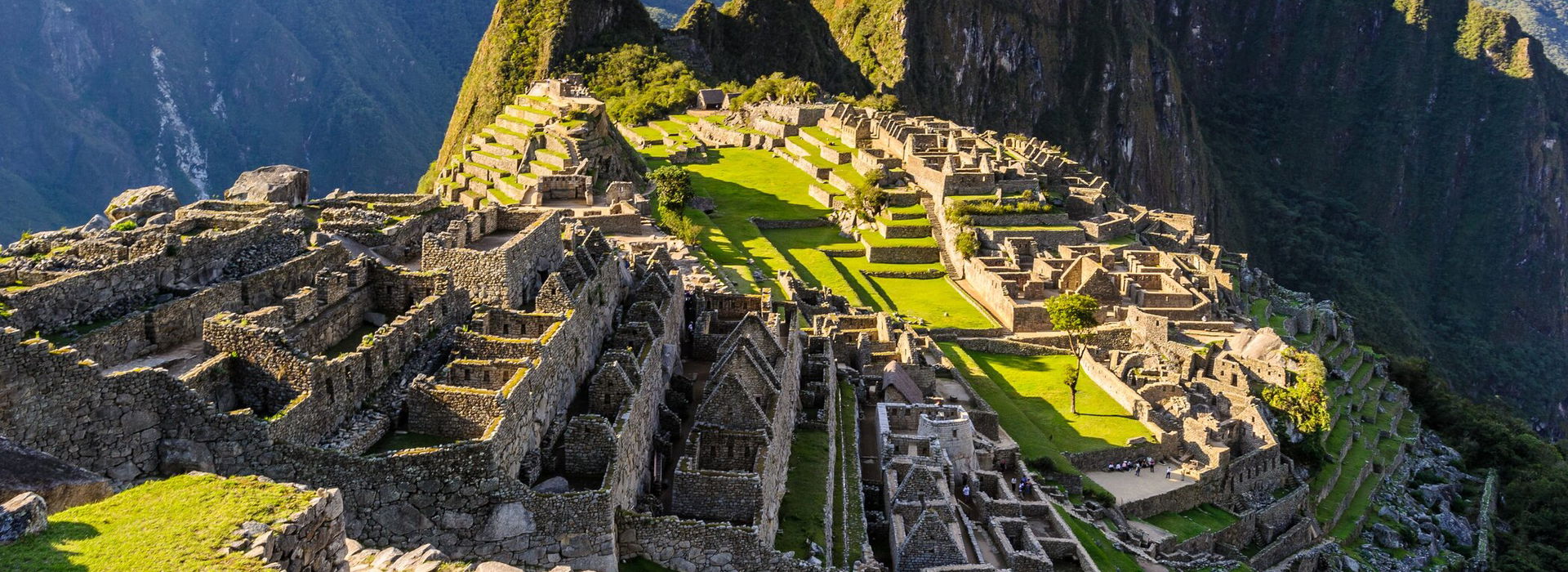The photograph captures an expansive and intricate aerial view of ancient ruins, likely reminiscent of Machu Picchu, sprawling across a mountaintop. The tiered and cascading structures are built from brown and tan stone, giving it a maze-like appearance that's visible due to the missing roofs. Surrounding walls and rooms stretch towards the upper left of the image, evoking a Pompeian style. Green grass and algae carpet the stone areas, which appear geometric and stair-like, adding vibrant patches to the scene under the sunlight. The ruins descend steeply into a deep canyon on the left and continue to cascade down into the valley to the right, emphasizing the verticality and grandeur of the site. In the background, mountains rise majestically, framing the location beautifully. Visible in the detailed image, the tiny figures of people highlight the immense scale and historical significance of these monumental ruins.